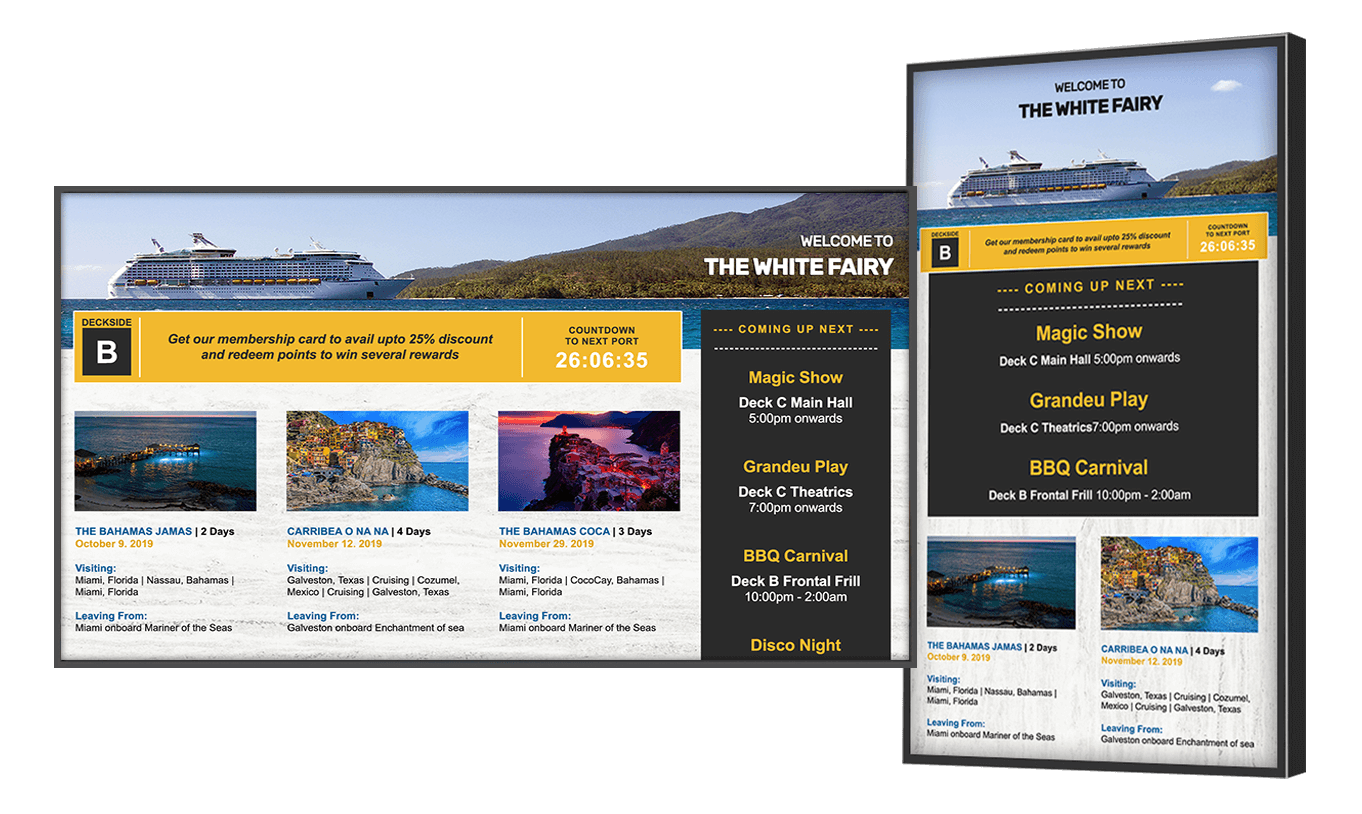The image comprises two rectangles: a larger horizontal rectangle and a smaller vertical one with a 3D appearance. Both rectangles feature a detailed photograph of a white cruise ship sailing on calm waters. The cruise ship, bathed in sunlight and shadows, has multiple floors and numerous windows, topped with a distinctive triangular structure. In the background of the image, lush, green-covered mountains stretch towards the water.

Beneath the ship's photograph, a yellow bar spans across both rectangles. On the left side of the bar, it reads "Deckside" next to a black square with the letter "B" inside. Adjacent to it, the text promotes a membership card offer: "Get our membership card to avail up to 25% discount and redeem points to win several rewards," though it should be noted that "upto" is incorrectly spaced. Below this, the text counts down to the next port with a timer showing "26 hours 6 minutes and 35 seconds."

The larger, horizontal rectangle also features a black vertical bar on the right side. At the top of this bar, in bright yellow font, are the words "Coming up next." Additionally, the image of the cruise ship includes the welcoming message "Welcome to the White Ferry."